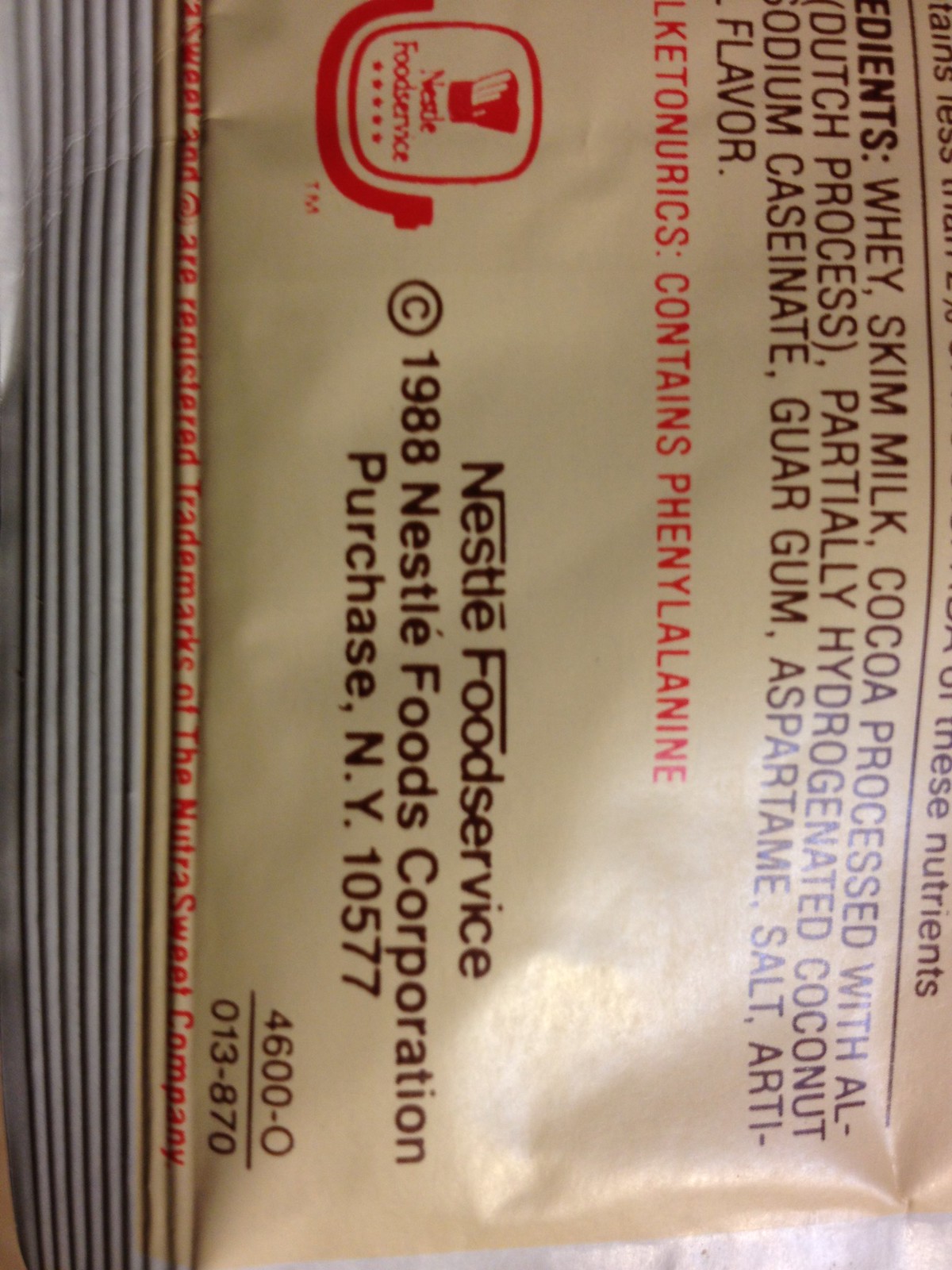A package, likely made of paper or plastic, is prominently displayed. The packaging lists ingredients that include whey, skim milk, cocoa processed with the Dutch process, partially hydrogenated coconut oil, sodium, cassonade, water, gum, aspartame, salt, and flavoring substances. Additionally, it mentions the presence of phenylalanine. Printed towards the middle left of the package is the text "Nestlé Food Service" along with an illustration of a chef's hat. In the bottom right corner, the copyright notice reads "© 1988 Nestlé Food Corporation." The company's address is listed as "Purchase, NY 10577." The package is sealed with crimps on the left side, and light is softly reflected on the bottom right of the image.